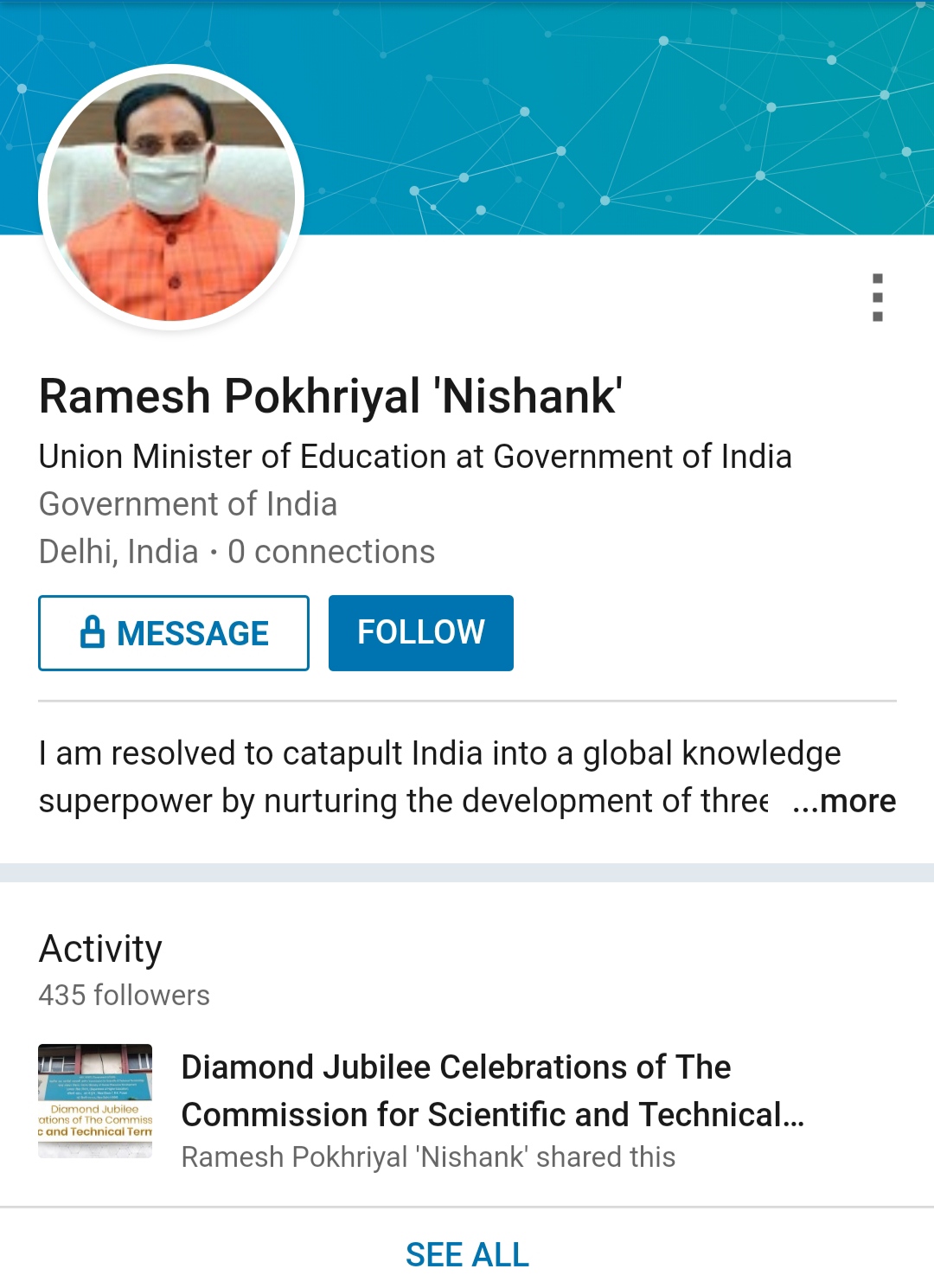This screenshot from a mobile app showcases the LinkedIn profile of Ramesh Pokhriyal 'Nishank', the Union Minister of Education for the Government of India. The profile is linked to the Government of India based in Delhi. The user looking at this profile has no mutual connections with Ramesh Pokhriyal. 

At the top of the profile, there is a simple blue banner followed by a circular profile image. In the image, Ramesh Pokhriyal is seen wearing a traditional sleeveless orange top with square patterns over a white buttoned-down shirt. He is also wearing a cloth mask.

The visible portion of Ramesh Pokhriyal's profile description states: "I am resolved to catapult India into a global knowledge superpower by nurturing the development of three..." followed by an option to read more.